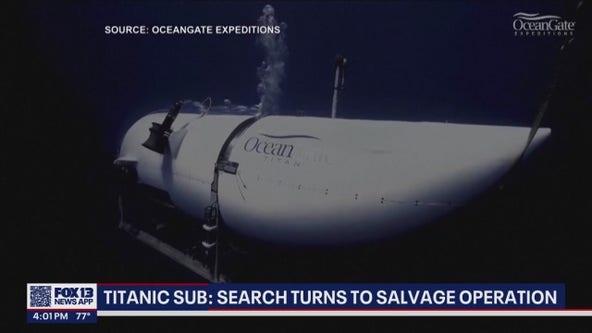This is an image captured from the Fox 13 News app, depicting an underwater scene featuring the OceanGate submarine that was lost several months ago. The screen displays various text overlays: in the top-left corner, white letters on a dark blue background read "Source: OceanGate Expeditions," and in the upper-right corner is the OceanGate logo. At the bottom left, it shows the time as 4:01 PM and the temperature as 77 degrees next to the Fox 13 News app logo. A banner on the right side announces in bold white letters, "Titanic Sub Search Turns to Salvage Operation," accentuated with a red-lined white strip underneath. The center of the image prominently features the white OceanGate submarine with light tan lettering spelling "OceanGate" on its side. The submarine is surrounded by a dark blue underwater backdrop, with air bubbles rising from its structure, indicating ongoing movement. The sub, pointed at one end with visible thrusters and a metal rack, is positioned as if descending into the depths.